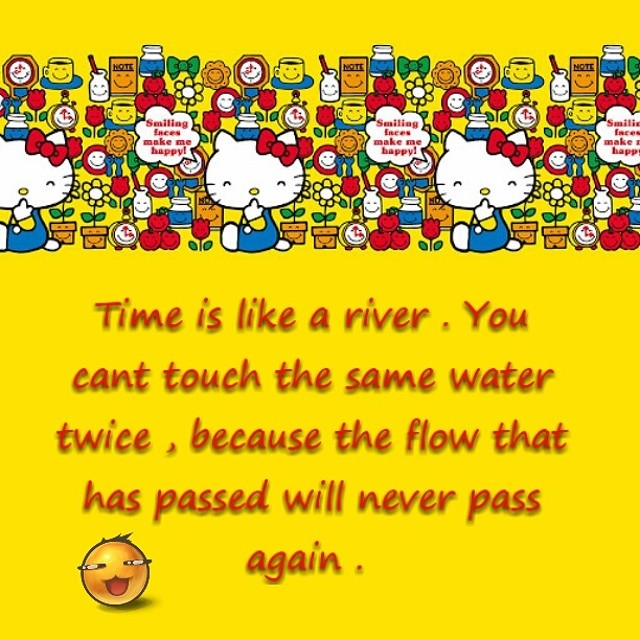The image features a vibrant, bright yellow background. The top third of the image is adorned with three cheerful white cartoon kittens, each with a red ribbon in their hair and dressed in blue coveralls. Surrounding the kittens are colorful elements such as potted flowers with smiley faces, white milk jugs with straws, yellow coffee cups on blue plates, and red flowers. The overall scene is lively and whimsical.

In the lower section of the image, there is a meaningful message written in red text: "Time is like a river. You can't touch the same water twice because the flow that has passed will never pass again." Adjacent to this text on the left side is a round smiley face emoji with slanted eyes, adding a playful touch to the profound message.

The detailed and colorful depiction, along with the insightful quotation, creates a captivating and thought-provoking visual.